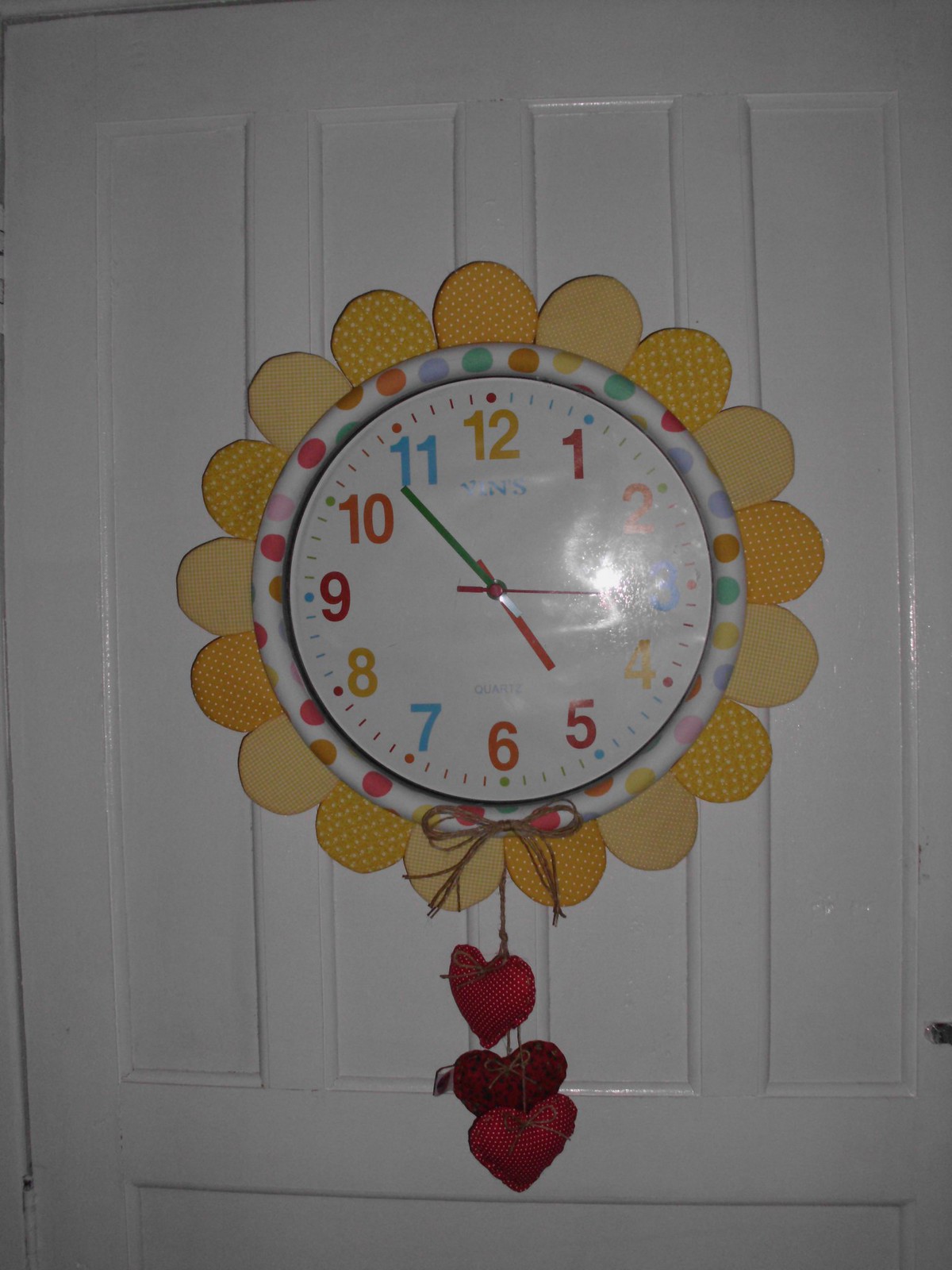This photograph features a whimsical analog clock affixed to the back of a white, interior residential door. The clock's dial is vibrantly painted, boasting a white background adorned with a playful array of multicolored polka dots. The numbers and ticks are similarly colorful, rendered in shades of red, blue, orange, and yellow. The clock's charm is further enhanced by an artistic frame of fabric leaves, mimicking the appearance of a sunflower's petals.

Adding to its quaint, country-cute aesthetic, the clock dangles three fabric puff hearts, each tied on with a rustic raffia string. This charming timepiece would make a delightful addition to a kitchen decorated in a traditional style or a cheerful touch to a child's bedroom.